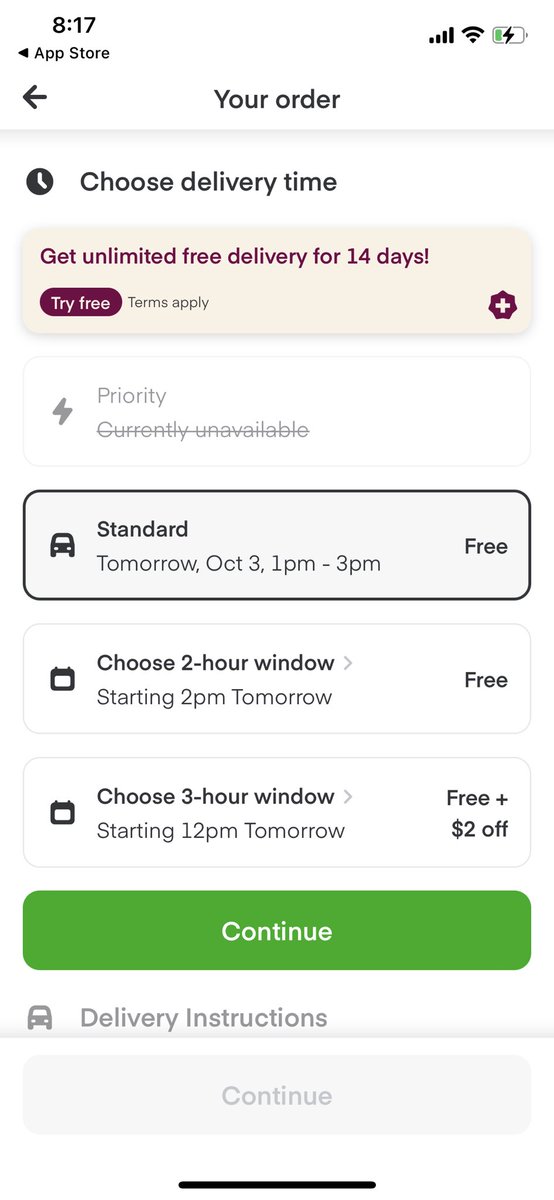Screenshot of a Mobile Order Delivery Page

The image is a screenshot of a cell phone displaying a delivery service application. The top of the screen features the status bar, showing the time as 8:17 AM, signal strength for internet connectivity, Wi-Fi indicator, and a battery icon.

Centered on the screen, the main heading reads "Your Order." To the left of this text is a back arrow icon. Below this, in bold black letters, is the prompt "Choose Delivery Time," encased in a rectangle with a light burgundy background and darker burgundy text.

Underneath, there's an offer outlined in a dark burgundy oval shape with white letters, reading "Get unlimited free delivery for 14 days." It also includes a "Try Free" button, with "Terms apply" noted in black text, adjacent to a circular emblem of a sun with a plus sign inside.

Following this, the options for delivery timings are listed:
1. **Priority (Currently Unavailable)** - This option has a line drawn through it, indicating unavailability.
2. **Standard** - Scheduled for tomorrow, October 3rd, between 1 PM to 3 PM, with a "Free" label.
3. **Choose 2 Hour Window** - Starting at 2 PM tomorrow, free of charge.
4. **Choose 3 Hour Window** - Starting at 12 PM tomorrow, also free plus an additional $2 off.

At the bottom, there is a prominent green rectangle with white text that reads "Continue." Below this, there is an area for delivery instructions and another "Continue" button in light grey, indicating an option yet to be activated.